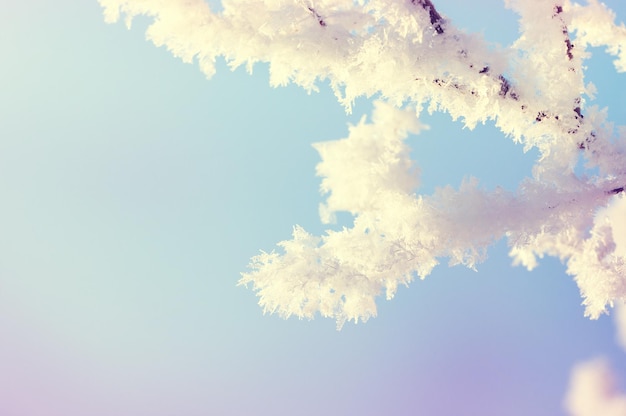The photograph showcases two main branches of a tree, delicate and serene, covered in pristine white ice crystals that shimmer in the sunlight. The background features a gradient of blue blending into purple at the bottom, providing a tranquil setting for the scene. Despite the lighting revealing the ice crystals distinctly, the wood of the branches is barely visible beneath the frosty coating, lending the branches a near cottony or feathery appearance. A part of the tree appears out of focus at the bottom, emphasizing the detailed form of the frosted branches and their fine offshoots. Lit from the left, the image captures the fragility of the ice-encrusted branches against the soft blue gradient, creating a calm, wintry aesthetic.